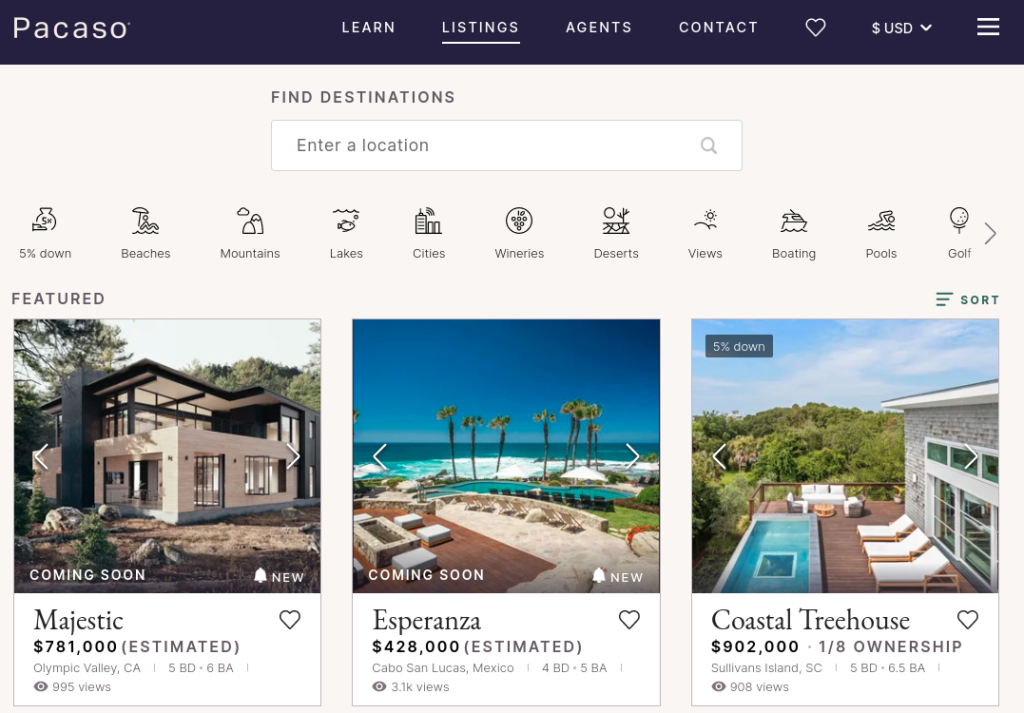In this detailed image of the PACASO website, "PACASO" is prominently displayed in white letters at the top left corner within a long blue navigation bar. This bar also features several menu options including "Learn," "Listings," "Agents," and "Contact." Additional icons in the navigation bar include a heart symbol, a currency selector labeled "USD" with a downward arrow, and a menu represented by three horizontal lines on the right-hand corner.

The central part of the page contains a search function within a white rectangular box that says, "Enter Location," underlined by the phrase "Find Destinations." Adjacent to this search box, there’s a section highlighting different types of destinations with icons and labels: "Beaches" (symbolized by a wave), "Mountains" (depicted by peaks), "Lakes" (shown with a fish in water), "Cities" (with a cityscape icon), along with others such as wineries, deserts, views, boating, pools, and golf. A right-arrow indicates more options are available.

Below this search area, the site displays a series of destination images labeled as "Coming Soon," each showcasing luxurious homes:

1. On the left, a picturesque property titled "Majestic" located in Olympic Valley, California. It features an estimated value of $781,000 and offers five bedrooms and six bathrooms.
2. In the center, there's a property named "Esperanza" in Cabo San Lucas, Mexico, valued at $428,000. This destination includes four bedrooms and five bathrooms.
3. To the right, a unique "Coastal Treehouse" home listed for $902,000 in Sullivan’s Island, South Carolina. This listing mentions one-eighth ownership and includes five bedrooms and 6.5 bathrooms.

These listings indicate options for partial ownership, suggesting that the platform offers luxury real estate share opportunities.